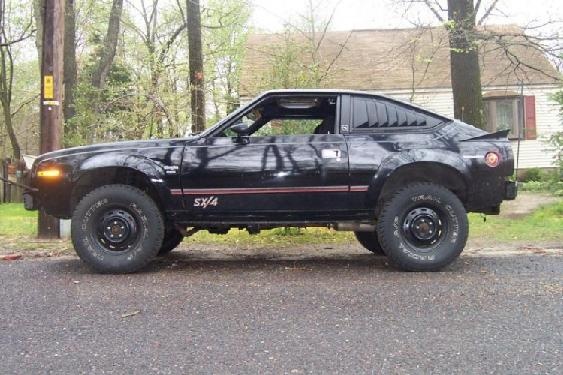A sleek, black sports car is parked on a smoothly paved street in front of a residential house. The car features distinctive black tires with white lettering, slightly blurred, and a striking red streak along the lower side, extending from wheel to wheel. The orange headlights add a contrasting detail, even though the car is viewed from the side. The vehicle appears to be a two-seater with its windows open, suggesting a sporty and aerodynamic design. In the background, a house stands amidst a lush landscape, featuring a manicured lawn, multiple trees with vivid green foliage, and a clear blue sky. A telephone pole is also visible, contributing to the suburban scenery.